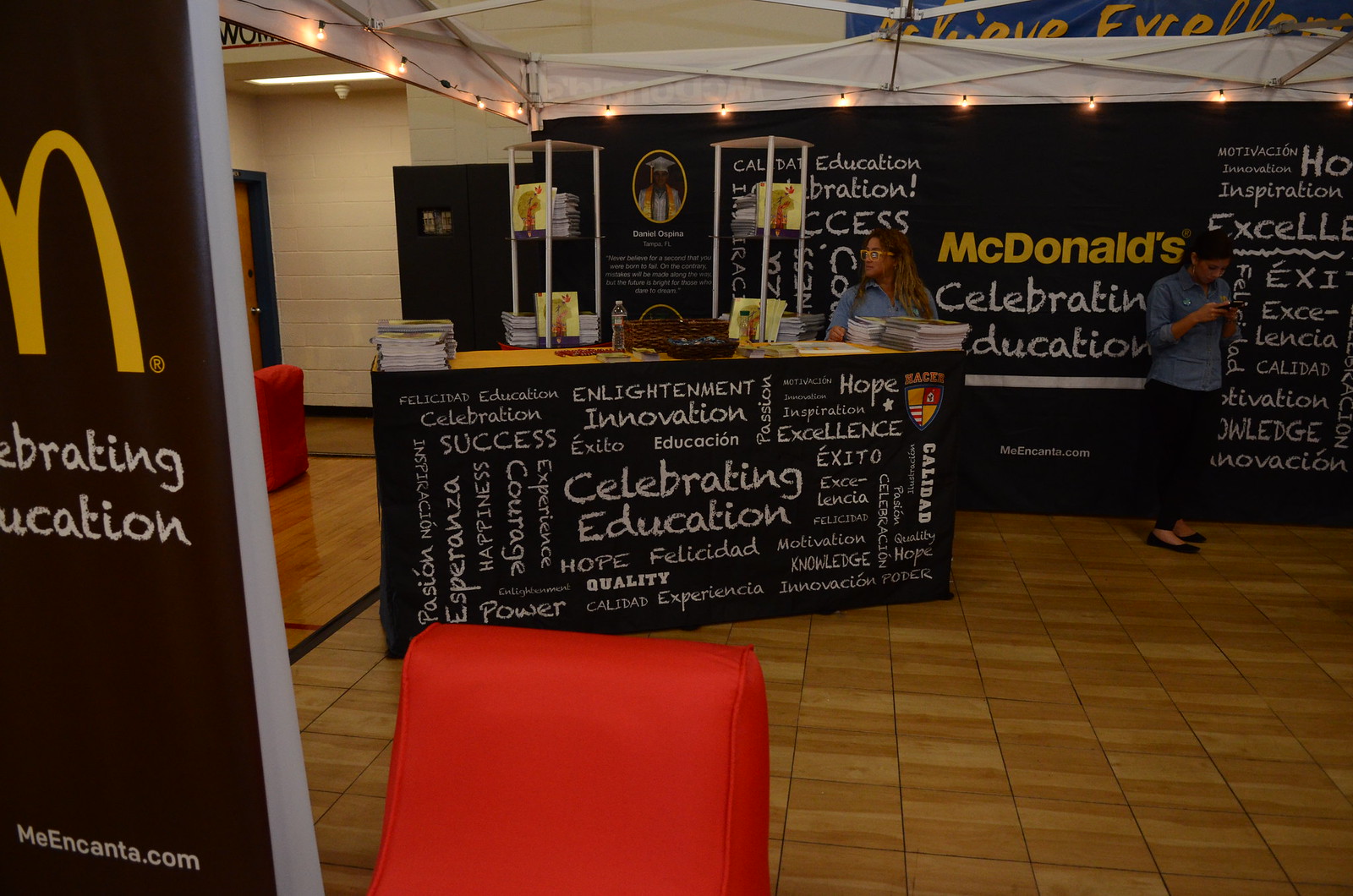The photograph captures an indoor scene that appears to be an event space, possibly sponsored by McDonald's. The setting features a brown tile floor and an array of orange and red cushioned seats. Central to the image is a long desk or podium, clad in a black sign festooned with white text that reads "Celebrating Education, Enlightenment, Innovation, Success," and topped with various books, pamphlets, and handouts. Behind the desk, a woman dressed in black pants and a blue shirt stands, while another similarly dressed woman stands to the side, focused on her phone. Both individuals appear to be part of the event staff. The backdrop includes black banners with McDonald's branding and inspirational words in white and yellow text, such as "Education," "Celebration," and "Excellencia". Overhead lights illuminate the setup, suggesting that the area is designed to catch the attention of passersby, possibly showcasing McDonald's involvement in educational initiatives. A glimpse of the iconic McDonald's arches can be seen, further emphasizing the brand's presence.